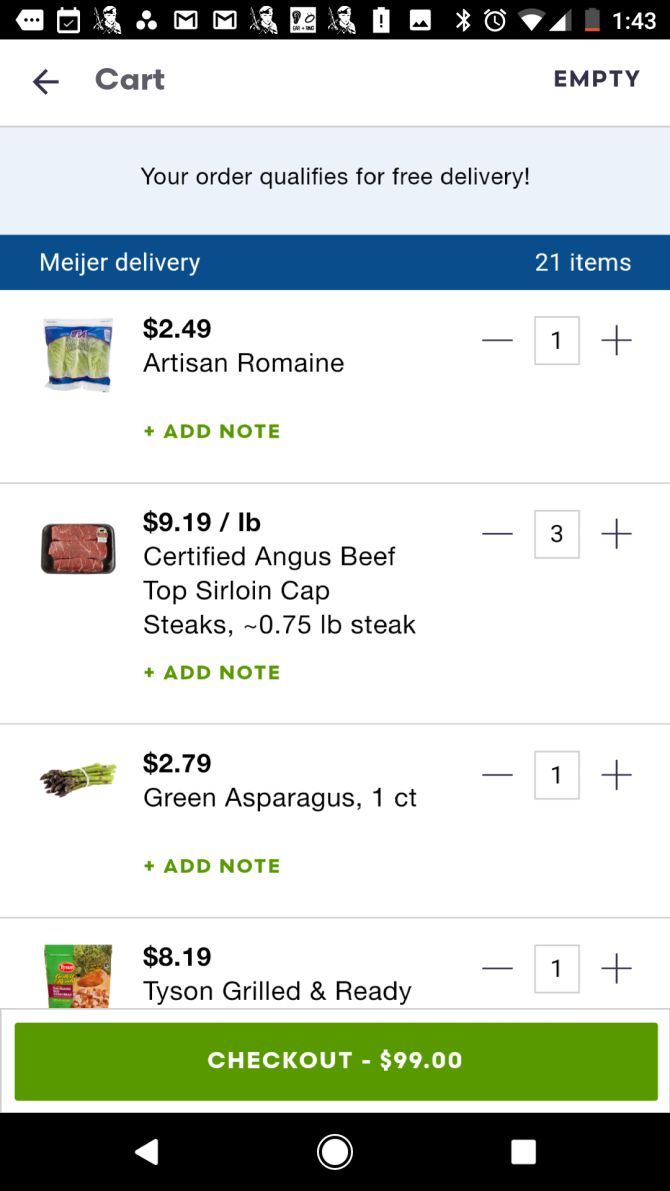The top section of the image displays a black bar containing various icons: a calendar, a person holding a gun, a trio of circles, a Gmail icon, another person holding a rifle, a white object, and a figure. Following this, there are several status indicators: a battery with an exclamation mark, a photo icon, a Bluetooth icon, a clock, nearly full WiFi signal, nearly full cellular signal, and a nearly depleted battery showing the time as 1:43 PM.

Below this, there seems to be a message or notification area with text reading: "Left or right of the car, empty, no order qualifies for free delivery, major delivery, 21 items, 249, artisan remain, 919, propellants, threading speed, top selling caps, 2.75 pounds, 2.79, green asparagus, 1 count, $10, $13, Tyson, Golden ready, minus 1 plus."

Further down, there is a green rectangle featuring "Checkout" and a price of $99. Lastly, the image includes navigation symbols in the form of a sideways triangle, a circle, and a square.